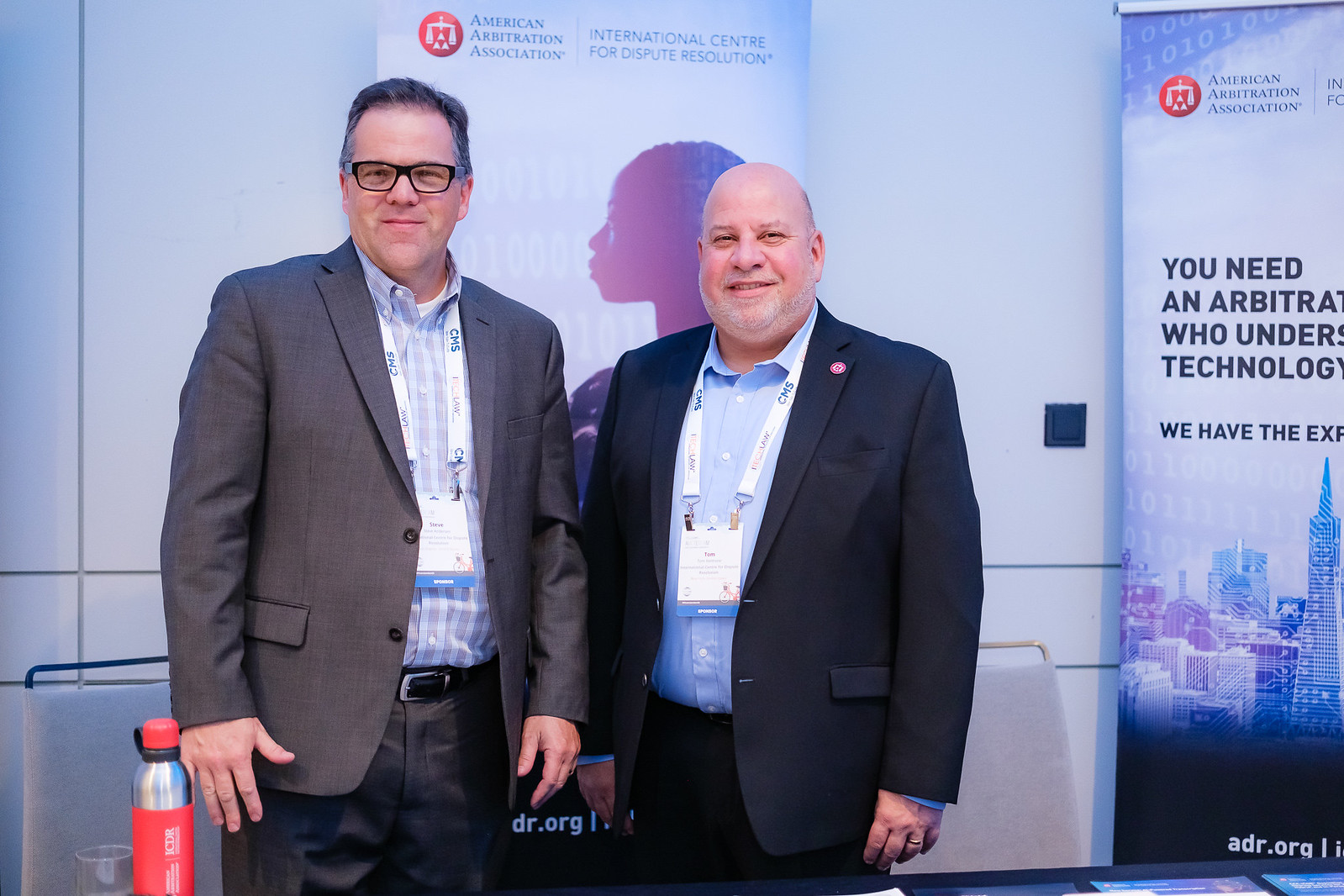This is a photograph of two older white gentlemen standing in front of a sign that reads "American Arbitration Association, International Center for Dispute Resolution." Both men are dressed in casual suits without ties, wearing white lanyards that display white rectangular cards with blue border letters. The gentleman on the left sports black rectangular glasses, short gray hair, a gray jacket, a blue dress shirt, and black pants. The man on the right is mostly bald with a large jaw, short stubbly white facial hair, a navy blue suit, and a blue shirt. The backdrop includes a red circle logo with white scales and features a printed cityscape image. Both men are smiling and posing for the camera, with a table of pamphlets visible at the bottom of the image.